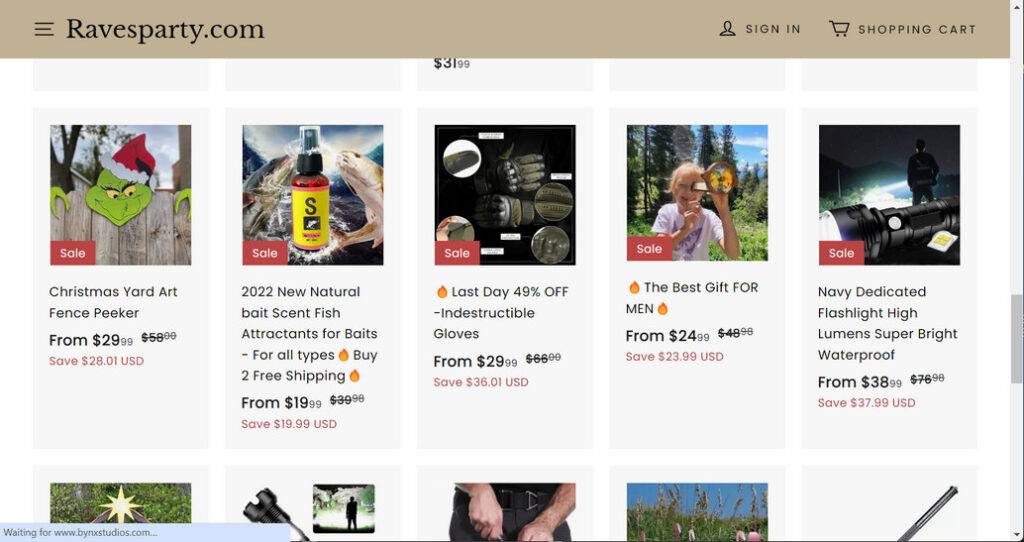The image depicts the homepage of a website called RavesParty.com, known for offering various products for sale. At the top of the page, there is a brown navigation bar. On the left side of this bar, the website's name, "RavesParty.com," is prominently displayed. On the right side, there are options to "Sign In" and access a shopping cart.

Below the navigation bar is a row showcasing five featured products. 

1. The first product on the left is an image of the Grinch peeking over a fence, marked with a "Sale" label in a red box at the bottom right corner. The text below the image reads, "Christmas Yard Art Fence Peeker from $29.99. Save $28.01 USD."
   
2. Next to it, there is a picture of a yellow and black bottle with fish images on either side. The description underneath states, "2022 New Natural Bait Scent Fish Attractants for Baits for All Types. Buy Two, Free Shipping from $19.99. Save $19.99 USD."

Though the exact details of the remaining three products in the row are not fully provided, their images are clearly visible, suggesting a variety of items available for purchase.

The partially visible row below indicates the presence of additional products, with the tops of five more items for sale just making it into the frame.